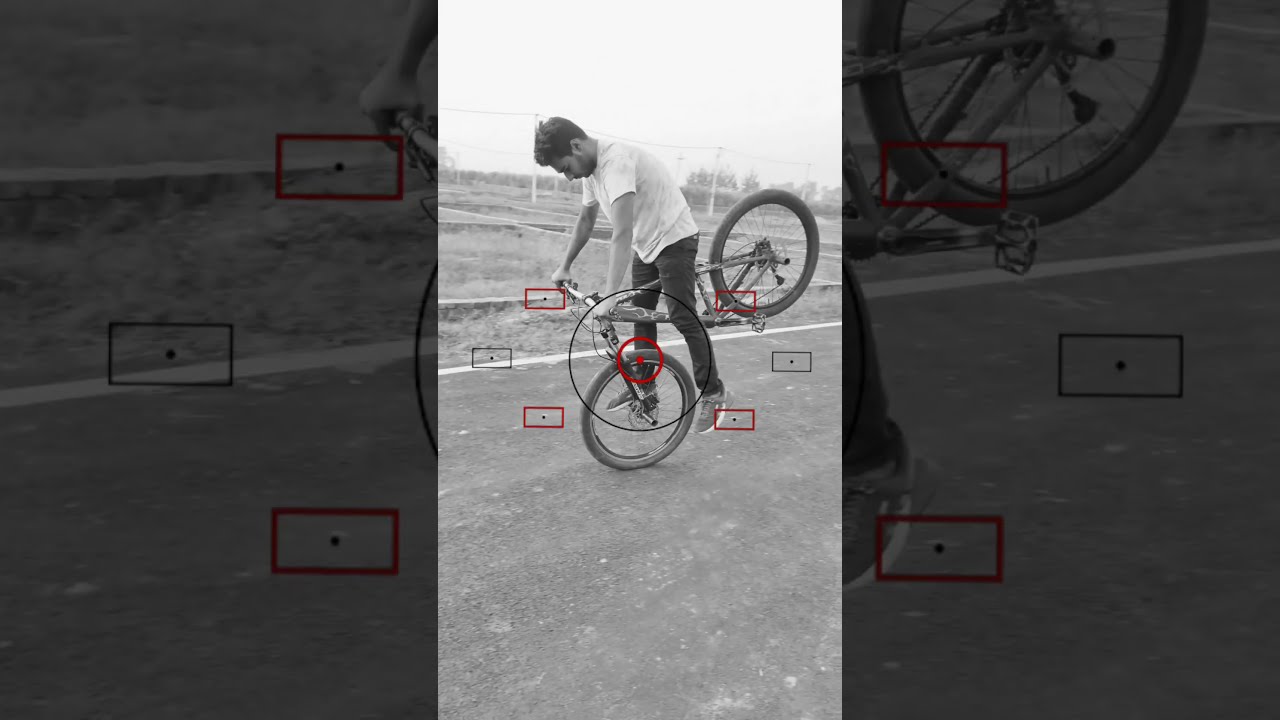A young man or late teenager with black hair, a beard, a white t-shirt, black skinny jeans, and dark sneakers is performing a bicycle trick on a BMX bike. In the black-and-white photo, he balances the bike on its front tire with the rear wheel lifted off the ground. He stands on the right peg of the front wheel, while his left leg hangs freely, aiding his balance. The backdrop appears to be an open field with a paved road surface underneath the bike. Overlaying the entire image are autofocus markings reminiscent of those seen through a professional camera lens. At the center is a black circle containing a red circle and a red dot. Surrounding the main circle are pairs of red and black squares, each with a corresponding black or red dot inside, mirroring the autofocus regions. Flanking the left and right of the photo are magnified versions of these squares.